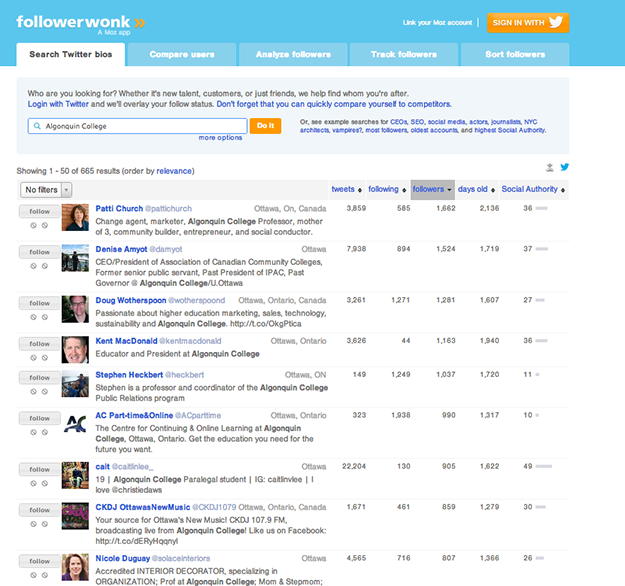The image showcases the interface of "Followerwonk," a Moz application. On the right side, there's an option to link your Moz account, accompanied by an orange "Sign in with Twitter" button featuring the Twitter logo. The interface is divided into five tabs: "Search Twitter Bios" (highlighted in white), "Compare Users," "Analyze Followers," "Track Followers," and "Sort Followers" (displayed in blue). Below these tabs, there's a search bar with an orange "Do It" button beside it. The area below the search bar displays a list of search results, showing 1 to 50 out of 665 results ranked by relevance. Each result includes a user's profile picture, their name in blue, and a brief description of who they are. Additionally, a chart is visible, listing metrics such as "Tweets," "Following," "Followers," "Days Old," and "Social Authority," with corresponding numerical values for each profile, ranging from low numbers to figures in the thousands.